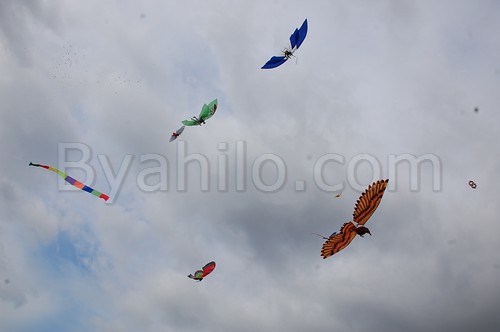The photograph captures a mostly cloud-covered sky with a small patch of blue peeking through in the bottom left corner. Floating in the sky are six kites designed to resemble birds, each varying in color and detail. The prominent bird-shaped kites include one that is blue and white, another green, an orange and black bird, and a brown and red bird with realistic-looking feathers visible on its wings. Additionally, there's a smaller red and green kite which appears less defined in shape, possibly resembling a dragonfly. Accompanying these is a unique kite that doesn't resemble an animal; instead, it looks like a colorful ribbon streaked with blocks of orange, pink, blue, red, and yellow. Across the middle of the image is the watermark "Biohilo.com."